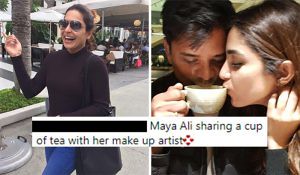The image consists of two side-by-side color photographs with some digital enhancement. The photo on the left is slightly out of focus and shows an outdoor scene with a smiling, dark-haired woman walking down a sidewalk. She is wearing sunglasses, a dark long-sleeved shirt, blue jeans, and carrying a purse. The background features planters with trees, umbrella tables, and possibly a restaurant setting. The text included in both pictures suggests that the woman on the left is Maya Ali.

The right photo depicts a young couple, a male and a female, both with dark hair, sharing a cup of tea. The setting appears to be indoors. There's a black rectangular banner at the bottom which reads "Maya Ali sharing a cup of tea with her makeup artist," implying that the woman in both photos is Maya Ali and the man in the right photo is her makeup artist. The colors in the image are vibrant and include shades of gray, blue, black, white, green, pink, and red. Despite the slight blur, the overall composition is clear and easy to understand.